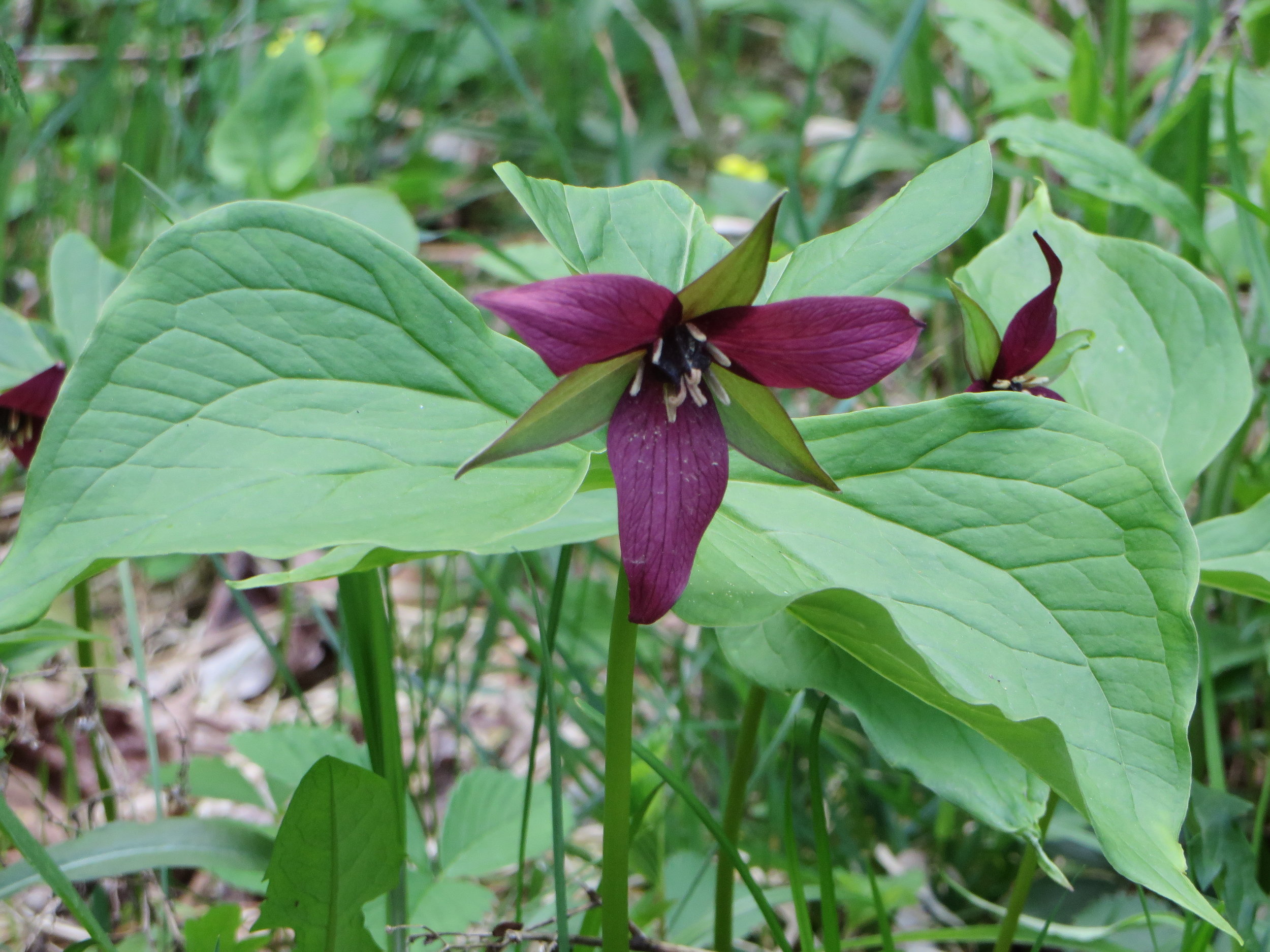The photograph captures a vibrant flowering plant in an outdoor setting. Dominating the foreground are large, teardrop-shaped leaves in a medium green shade, punctuated by a prominent center vein and numerous smaller veins. These large leaves frame a striking purple flower at the center, which boasts three elongated purple petals adorned with dark purple veins. Between each purple petal, there are three pointed green leaves, creating a pattern that alternates between purple and green. Emerging from the flower's core are black stamens tipped with white. To the right, another similar purple flower is visible. The background is blurry but suggests an abundance of green stems and hints of yellow flowers, complemented by the earthy tones of branches, dead plant matter, and brown leaves on the ground below, indicating an outdoor environment.